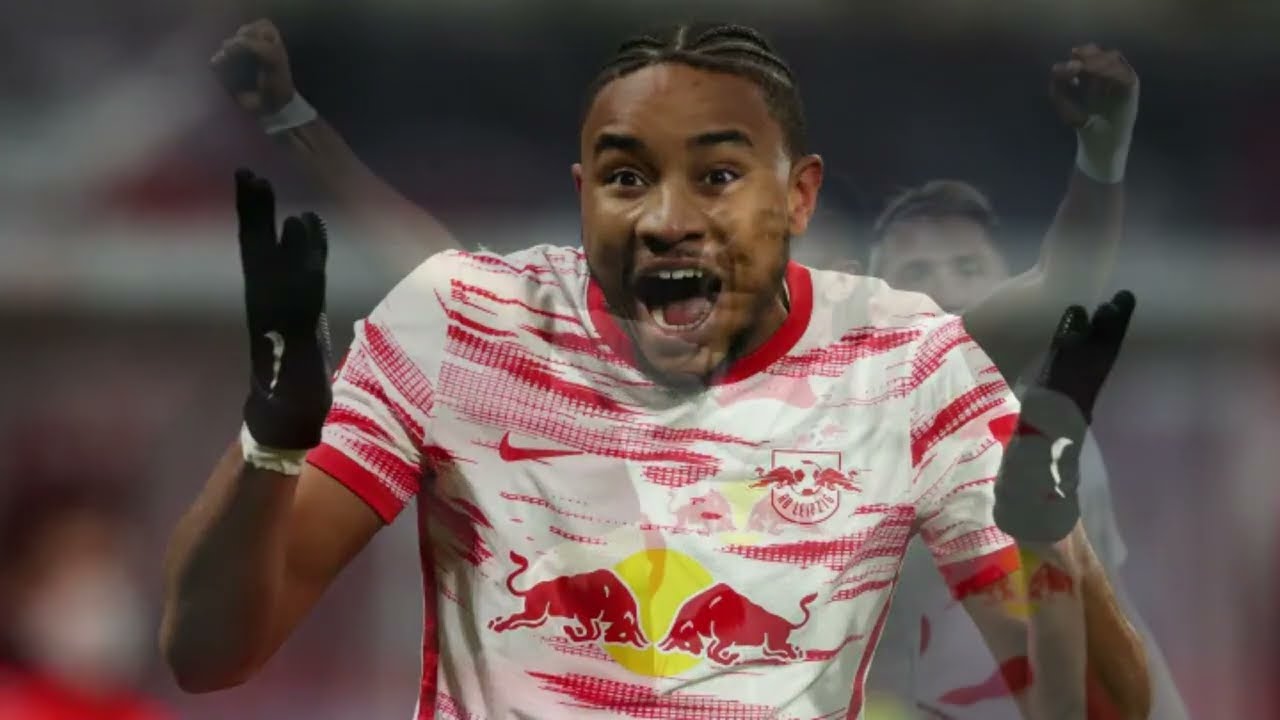The image depicts an African-American soccer player, likely from the New York Red Bulls, in a moment of high emotion, possibly celebrating a goal. He is positioned at the center of the shot, visible from the torso up, with his arms extended outwards and elbows bent, hands lifted towards the sky. He is wearing black Nike gloves, a red and white jersey featuring the Red Bull logo prominently on his chest, and a tightly worn hood over his cornrow hairstyle. His mouth is wide open, suggesting a scream or shout of joy.

Behind the main figure, there are two superimposed, semi-transparent images of other players. One appears to be a Caucasian individual in a white shirt, also in a celebratory stance with arms raised. The second figure, possibly in a long-sleeved shirt, has clenched fists in the air. These background figures are only partially visible, maintaining a primary focus on the ecstatic main player in the foreground.